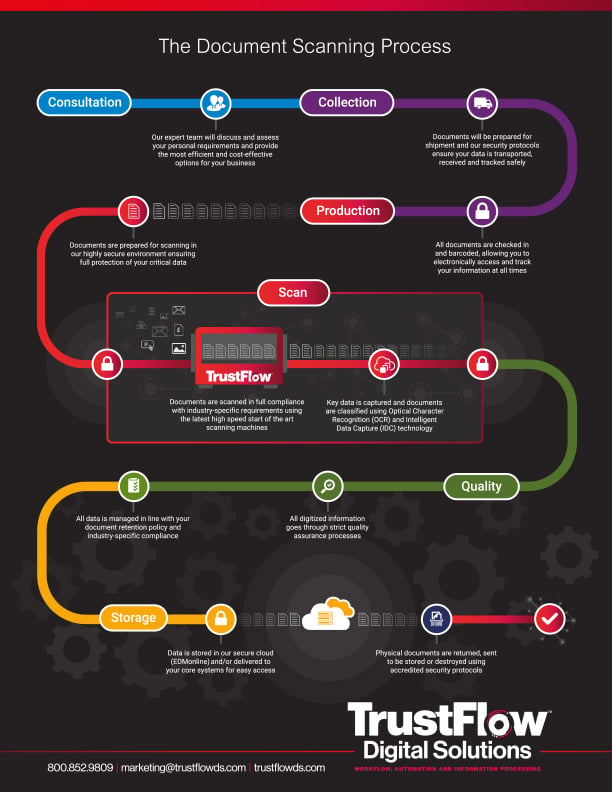This detailed flowchart from TrustFlow Digital Solutions illustrates their comprehensive document scanning process against a striking black background, enhanced by colorful segments and clear step-wise distinctions. 

Starting at the top left, the initial blue section labeled "Consultation" involves a thorough discussion and assessment of your specific requirements by the expert team to provide the most efficient and cost-effective options. Following this, a blue line leads to the “Collection” stage, marked by a purple segment and a truck icon, where documents are prepared for shipment under stringent security protocols, ensuring safe and transparent receipt and tracking.

The flow then transitions to a red-line pathway into the “Production” phase, which houses a secure environment for document processing. Here, documents are checked in, bar-coded, and scanned using OCR (Optical Character Recognition) technology to capture and classify key data in compliance with industry requirements.

As the red line curves around the chart's margin, it intersects with “Quality” in a green segment. This stage ensures all digital data undergoes strict quality assurance processes and is managed in alignment with document retention policies. Subsequently, the pathway turns yellow and leads to “Storage,” marked by a cloud icon indicating the secure storage of data in the cloud.

Finally, the colorful flow concludes at the bottom right of the chart with a red checkmark, symbolizing the return or secure destruction of physical documents according to accredited security protocols. At the bottom of the flowchart, TrustFlow Digital Solutions’ logo is displayed, alongside their contact details: phone number 800-852-9809, email marketing@TrustFlowDS.com, and website TrustFlowDS.com, emphasizing their expertise in automation and information processing.